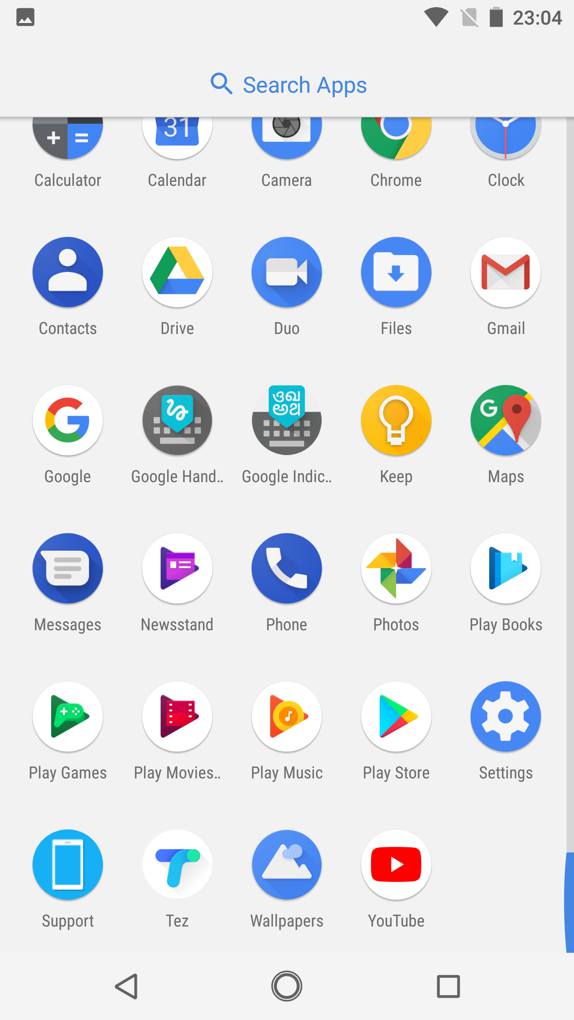Here's a refined and detailed caption for the image based on the provided description:

---

The image depicts an Android app drawer with a predominantly light gray background. The app icons are styled uniformly with circular outlines, creating a consistent and streamlined visual theme. The visible apps include a mix of basic and additional utilities, listed as follows: Calculator, Calendar, Camera, Chrome, Clock, Contacts, Drive, Duo, Files, Gmail, Google, Google Handwriting Input, Google Keep, Maps, Messages, Newsstand, Phone, Photos, Play Books, Play Games, Play Movies, Play Music, Play Store, Settings, Support, Tez (an app for digital payments), Wallpapers, and YouTube. Some Google apps are present but not easily identifiable, possibly for hand gestures or other functionalities. The battery indicator shows a full charge, and there are potentially more apps above the current view if the screen were scrolled up.

---

This caption aims to give a detailed and structured overview of the app drawer's content and aesthetic features.